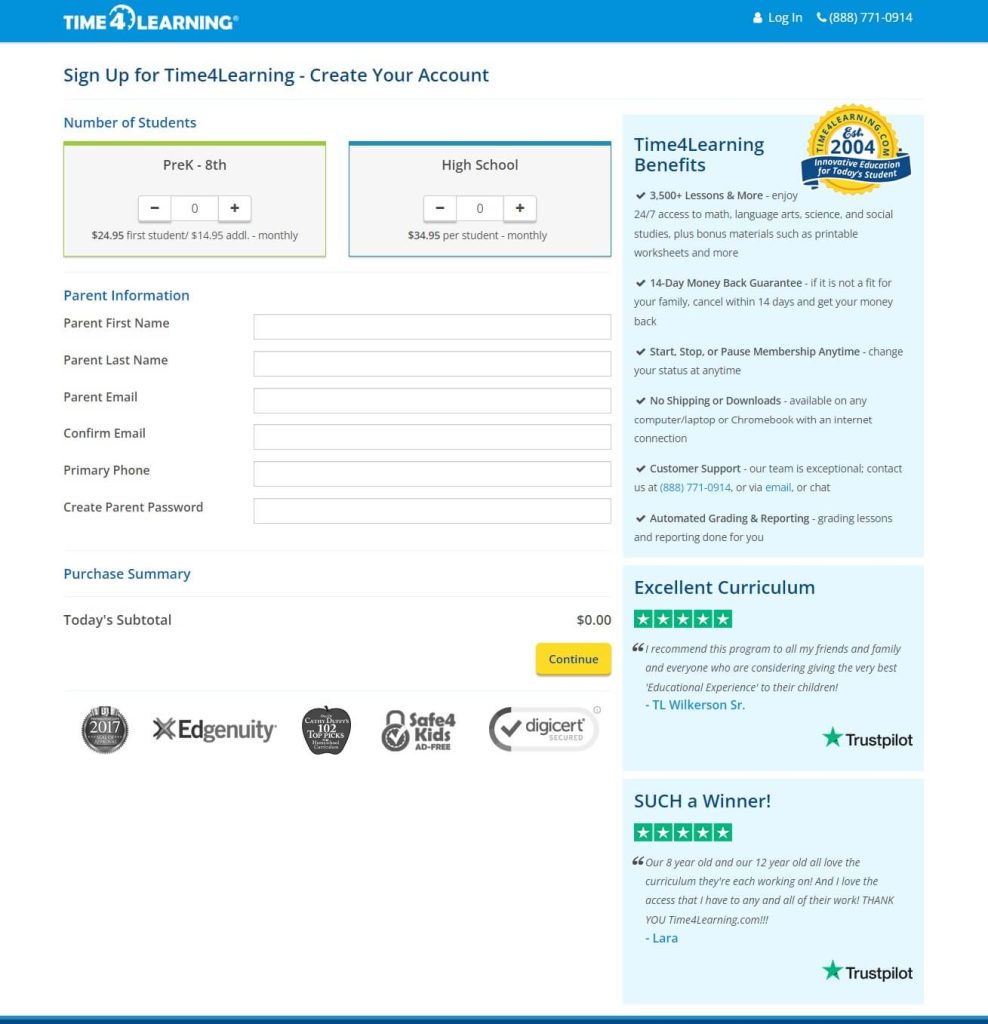A detailed view of a website registration form for a learning platform. The center showcases a form with relevant information surrounding it. At the top, enclosed in a blue border, the text reads "Time for Learning," accompanied by a login option and a contact phone number, 888-771-0914, in the upper right corner. Below, users are encouraged to sign up for "Time for Learning" by creating an account. The form includes sections to select the number of students: for Pre-K through 8th grade, priced at $24.95 per student with an additional $15 monthly fee, and for high school students, priced at $34.95 per student per month.

The parent information section requires details such as the parent's first name, last name, email address (with confirmation), primary phone number, and the creation of a parent password. The purchase summary indicates a current subtotal of zero, with a button labeled "Continue" for proceeding to the next step.

Various icons at the bottom display certifications and rewards, such as "Safe for Kids," "Ad-Free," "Edgenuity," and "DigiCert Secured." On the right side of the page, highlighted benefits of "Time for Learning" are listed, including access to 3,500 lessons, 24/7 availability for subjects like math, language arts, sciences, and social studies, along with bonus printable worksheets. Additional features mentioned are a 14-day money-back guarantee, the flexibility to start, stop, or pause membership anytime, no shipping or downloads required, customer support, automated grading and reporting, and the high quality of the curriculum, supported by two five-star reviews on Trustpilot.